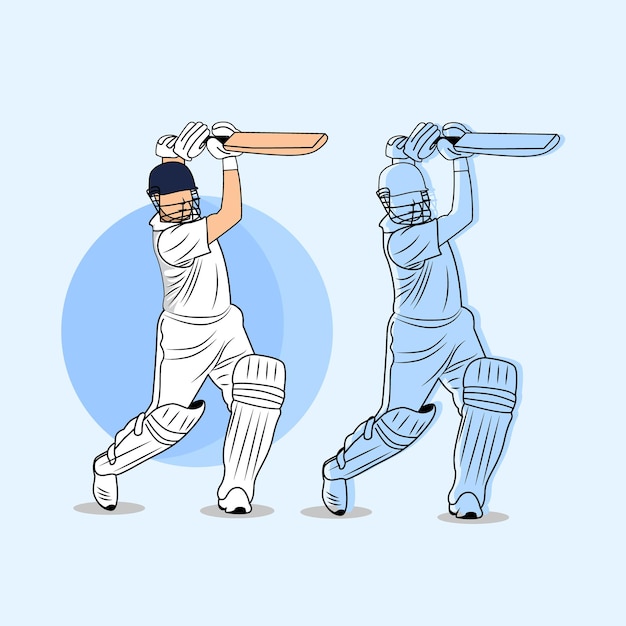The illustration features two side-by-side cricket players in identical poses, swinging their bats as if they've just hit a ball. The player on the left is depicted with realistic colors, showcasing a flesh-toned arm and head, wearing an all-white cricket uniform, including a shirt, pants, leg guards, shoes, and gloves. He also sports a black helmet with a face guard and holds a brown cricket bat. In contrast, the player on the right is entirely in shades of blue, appearing more stylized and abstract. The artwork is set against a light teal or mint blue background, with two overlapping circles behind the player on the left, one dark blue and one light blue, similar to a Venn diagram. Both players are facing the viewer with their torsos twisted and right arms raised, holding the bat parallel to the ground.